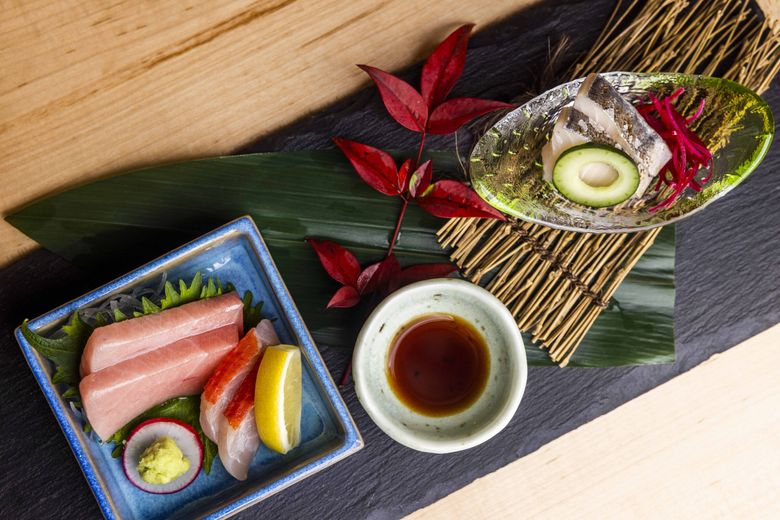A beautifully arranged, natural-looking platter of food is presented on a wooden table, making for an exquisite and healthy meal display. Central to the composition is a square blue plate featuring neatly arranged thick slices of fresh fish, likely salmon, accompanied by two smaller pieces of another type of fish. The fish slices rest on a bed of vibrant green lettuce. Adding a touch of sharpness, a small wedge of lemon is placed beside a radish slice topped with a dollop of wasabi or a similar green condiment.

To the right of the blue plate, a small white bowl filled with soy sauce is set, the bowl and plate both situated on a wide, dark green palm frond. This palm frond lies across a mat that appears to be woven from small twigs, designed with intricate craftsmanship. A striking red sprig, likely decorative, adds a splash of color to the arrangement.

Another intricate detail includes a shell containing slices of cucumber and possibly beetroot placed on the left side, enhancing the visual and textural variety of the dish. This, too, rests on the wooden table, which serves as a warm and rustic backdrop to the elegant presentation. The overall setting, complete with a light-green and yellow painted glass plate propped on the twig mat, evokes a sophisticated yet natural dining experience, making it worthy of a feature in a high-end cooking magazine.